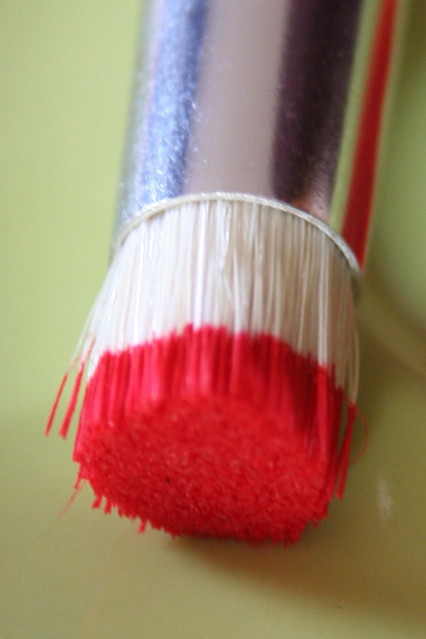This highly zoomed-in image captures the end of a paintbrush with meticulous detail. The focal point is the silver metal ferrule that secures the white, dense, and short bristles to the handle. The ferrule exhibits reflections of blue, red, and green light, with the green being a reflection from the surface the brush rests upon. A clear red stripe of paint adorns the tip of the bristles, vividly contrasting with their white color. The entire scene rests on a light olive green background, adding a subtle hue to the reflections on the metal. Additionally, a few bristles protrude slightly from the otherwise neatly clumped arrangement, enhancing the intricate details of the brush captured in this close-up shot.